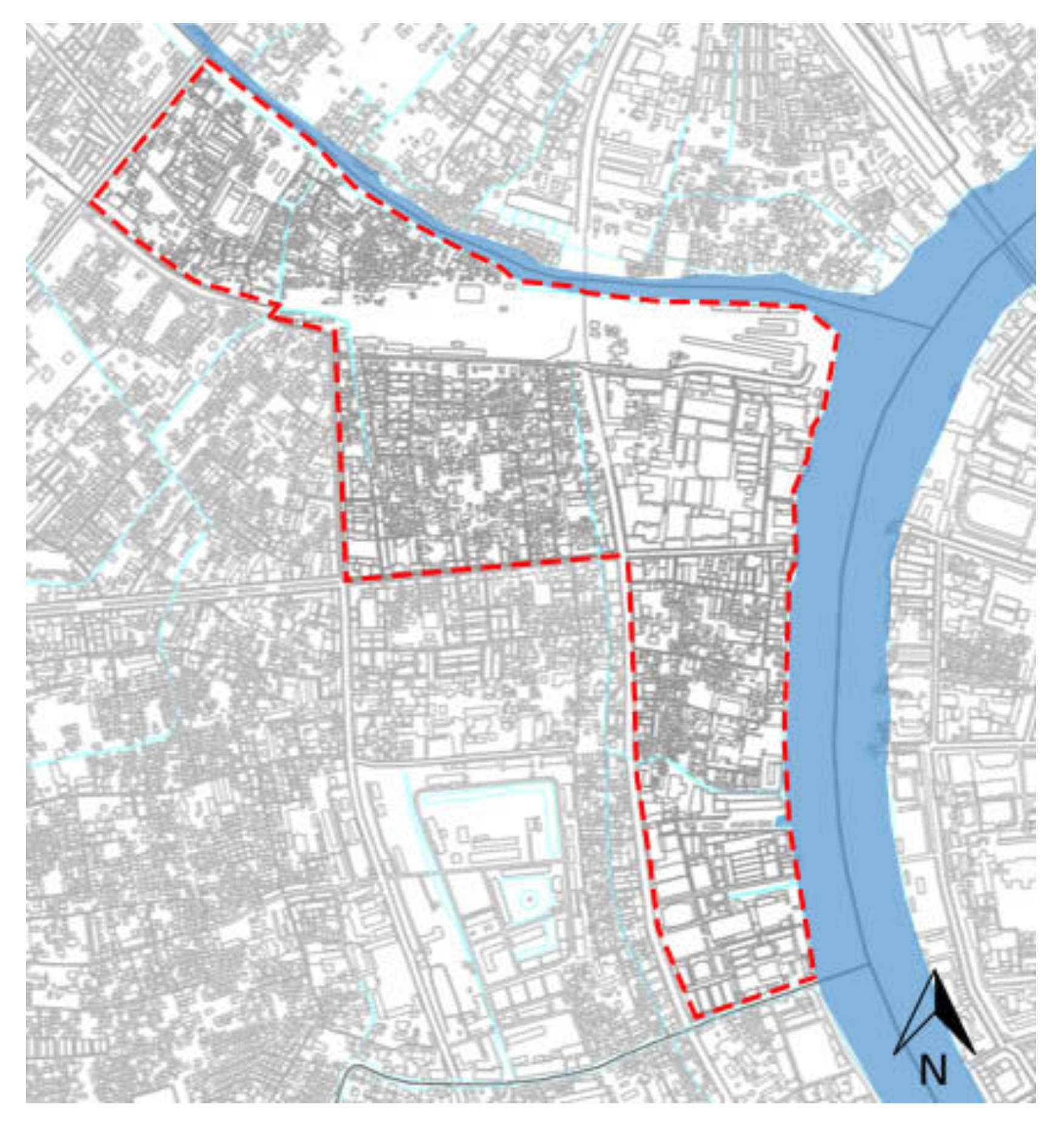This drawn map displays a detailed aerial view with a light gray and white background. A prominent feature is the river highlighted in blue, curving from just below the upper right corner down to the bottom right. From this main river, a much thinner tributary branches off, extending towards the upper left corner. A distinctive red-dotted line encircles a gun-shaped area on the left-hand side of the river, encompassing a section that runs along the lower part of the tributary and river. Additionally, at the bottom right corner, there's an arrow-shaped directional emblem that indicates north, with its right side in black and its left side transparent, through which the river is visible. The overall layout includes no visible street or city names, but clear geographical delineations and a distinctive upside-down L or foot-like area define the central map section.